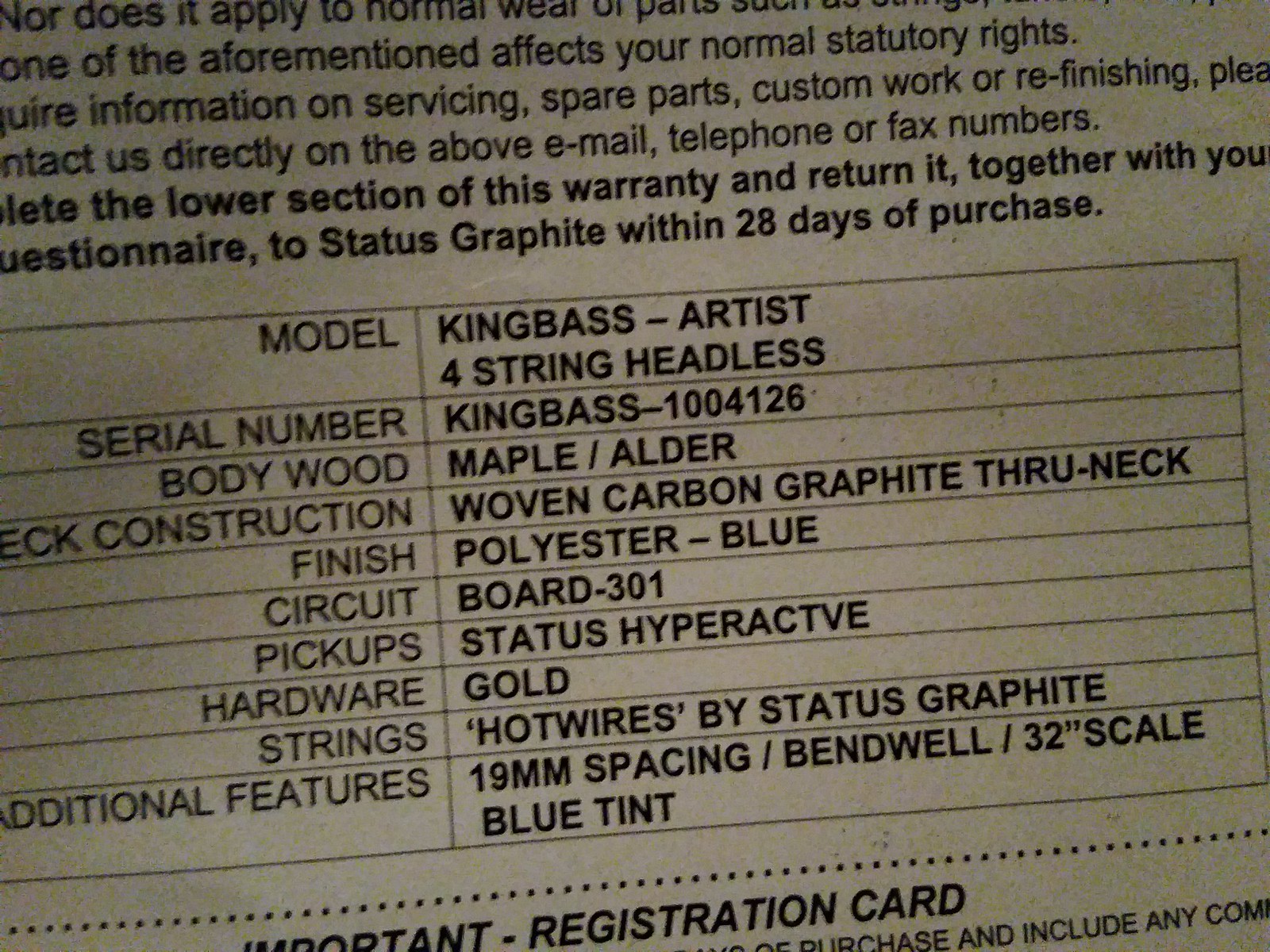This is a detailed black and white image of a label, likely a guitar warranty and registration form. The visible text starts with a partial statement, "nor does it apply to normal wear, or maybe it says parts, such," followed by a cut-off word. The next legible line reads, "one of the aforementioned affects your normal statutory rights." Subsequent lines provide information on "servicing, spare parts, custom work, or refinishing. Contact us directly on the above email, telephone, or fax numbers." Below this, it instructs to "complete the lower section of this warranty and return it together with your questionnaire to Status Graph within 20 days of purchase." 

Additionally, it features detailed specifications of a guitar model labeled "King Bass Artist, Four String Headless," with the serial number "King Bass 1004126." The guitar's body is described as wood with a maple outer and a woven carbon graphite through-neck construction, finished in polyester blue. It includes a circuitry board labeled "301," Status Hyperactive pickups, and gold hardware. The strings are identified as "Hot Wires by Status Graphite," and it features 19mm spacing, a bend wheel, and a 32-inch scale with a blue tint.